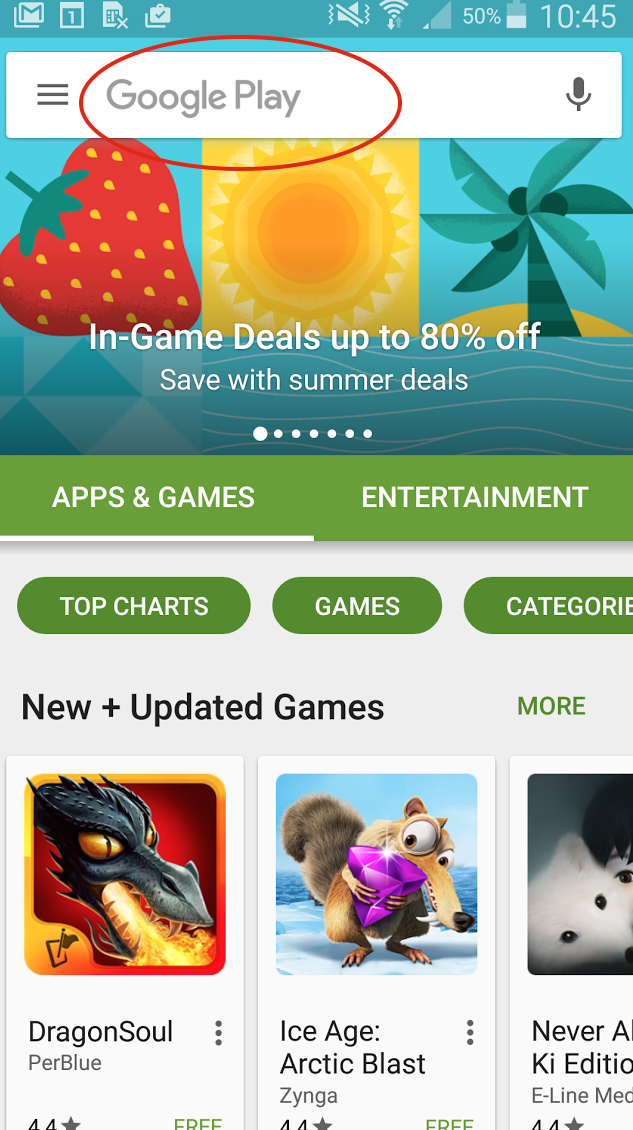The image depicts a digital screen with a predominantly teal-colored theme. At the very top, there is a teal-colored search bar labeled "Google Play," featuring a gray and red circle icon. To the left of the search bar, there are three gray lines, representing the menu icon, and above it, a gray microphone icon.

Below the search bar, there is a status bar displaying various icons in white: an 'M' likely representing Google Mail, a calendar icon with the number one, a vertical line, an 'X' icon, and a briefcase. This bar indicates the phone's battery level, showing it is 50% charged, alongside the current time, 10:45.

Beneath the status bar is the main content area, starting with a highlight section for Google Play showing a red strawberry icon with yellow seeds and a green top. Next to it is a yellow sun-like icon, and a teal-colored tree below it. This is followed by a promotional banner in white text stating, "In-game deals up to 80% off. Save on some of these deals."

Below the promotional banner, there are various navigation tabs. The left side features "Apps & games" in yellow, underlined to indicate the currently active section, and the right side displays "Entertainment."

Under these tabs are three green ovals with white text: "Top charts," "Game categories," and another oval, each outlining different sections of the app store. Below these, in black text, the section title reads "New + updated games," with a green "More" button adjacent to it.

Three game listings are partially visible underneath:
1. "Dragon Soul" features a purple-blue theme, a rating of 4.4 stars, marked as free, and includes an image of a black dragon.
2. "Ice Age: Arctic Blast" displays a rating of 4.4 stars, marked as free, with an image of a squirrel holding a purple diamond.
3. "Never Alone: KI Edition" shows a partially visible title, a rating of 4.4 stars, and an image of a white dog.

This comprehensive layout vividly portrays a snapshot of the Google Play Store's user interface, particularly highlighting ongoing deals, new and updated games, and navigation options.